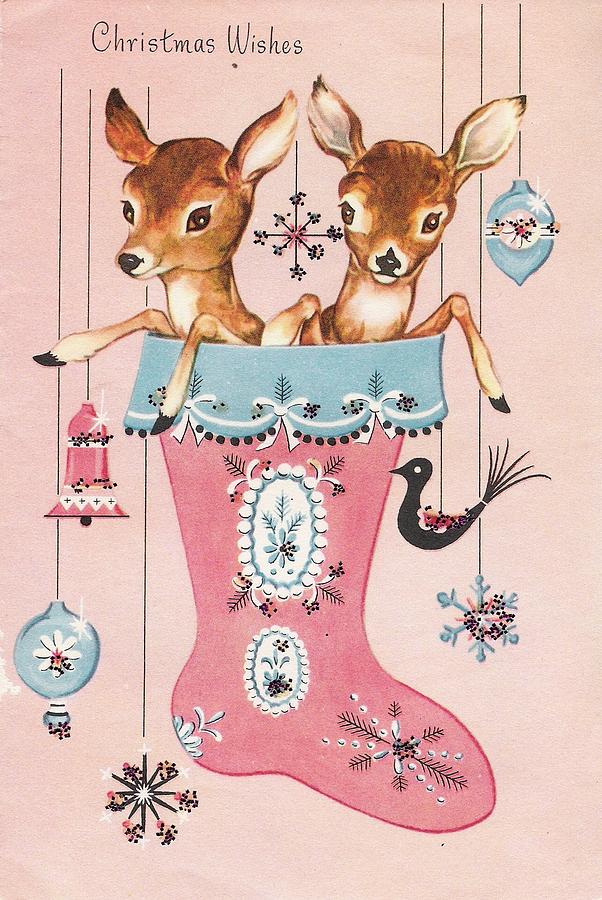This charming Christmas card features a light pink background with the festive greeting "Christmas Wishes" at the top. Hanging from black strings are various ornaments, including pink and blue bells, delicate blue and pink snowflakes, and a small black bird. At the center of the card is a pink stocking with blue lace trim and adorned with three white bows and additional white decorations. Inside the stocking are two adorable baby deer, tan and white with bright eyes and perky ears, peeking out with their little hooves dangling over the side. Their innocence and cuteness are highlighted by the snowflake nestled between them. The card's color palette is a cheerful mix of pink, blue, black, tan, and white, creating a warm and festive scene.